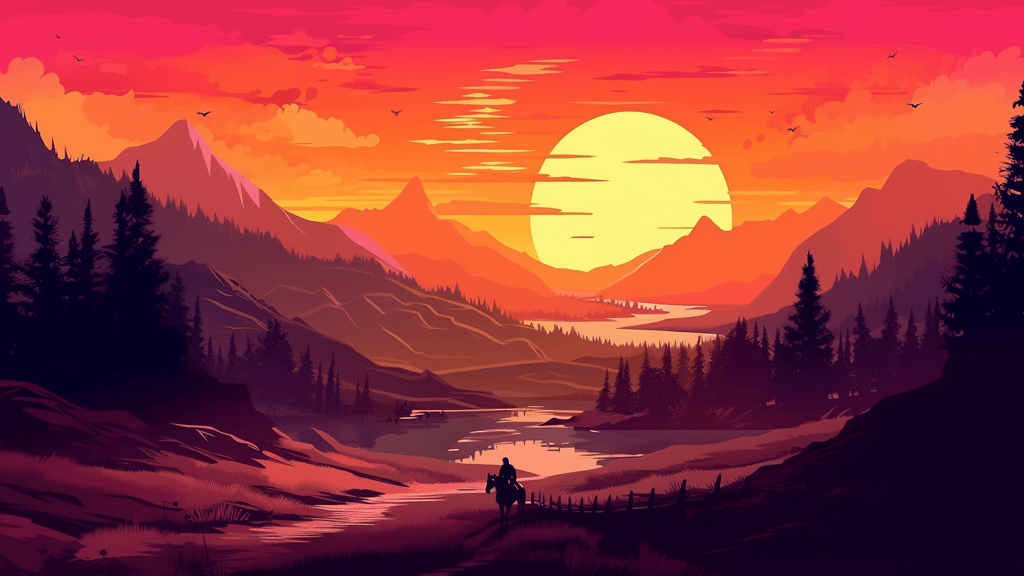The image is a richly detailed, digitized computer graphic of a dramatic sunset over a canyon-like mountain range reminiscent of the Grand Canyon. The backdrop is dominated by jagged peaks in shades of eggplant and light purple, interspersed with silhouettes of trees. Central to the scene is an enormous, light yellow sun, casting a romantic red hue across the landscape, flanked by clouds tinted with orange, pink, and magenta.

In the foreground, a small silhouette of a person on horseback stands by a serene lake off a rough trail, adding a western touch to the scene. The winding river snakes from the bottom center of the image up to where it disappears into a distant valley beneath the setting sun. Snow-capped mountains rise on either side of the scene, completing this picturesque and evocative landscape.